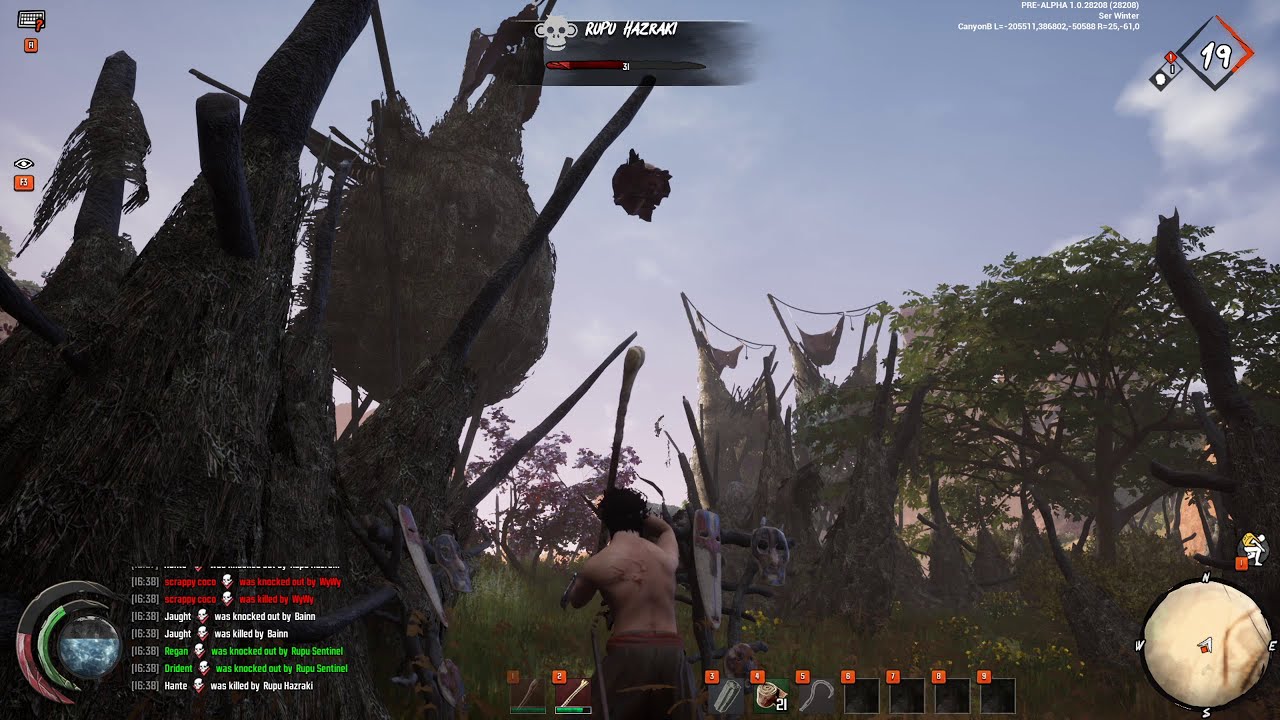This image is a detailed screenshot taken from a video game depicting an outdoor scene under mostly clear, blue skies with a few clouds on the right. The top middle displays the name "Rupu Hazuraki" along with a half-depleted red health bar. On the top right corner, a black and orange triangle shows the number 19.

The middle front of the image features a shirtless man with black hair, seen from behind, appearing to hang masks on a wooden fence-like structure. He holds a long staff and wears a brownish skirt. Surrounding him is an environment characterized by grass, green-leaved trees, and what appears to be a fort or various wooden structures resembling teepees. These structures hold masks and shields.

On the bottom left corner, there are green or brown blocks with small orange sections in their top left corners, possibly representing in-game items or events. Additionally, the game chat and a stamina bar in the form of a circle with two crescents are present. On the bottom right corner, there is a circular map displaying cardinal directions with the character's icon as a white triangle pointing north.